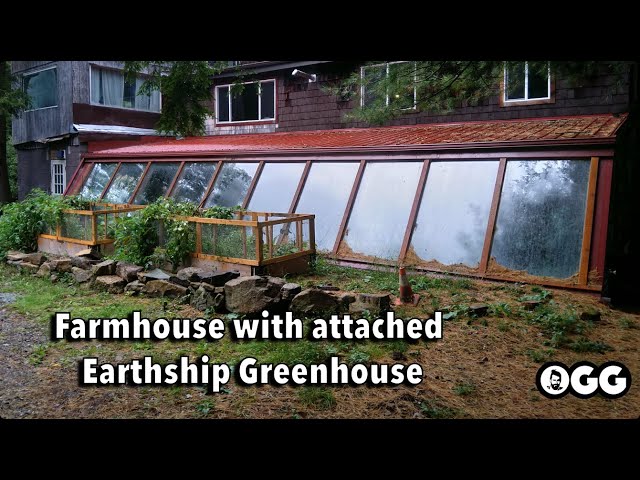This horizontal photograph captures a detailed view of a wooden greenhouse attached to a farmhouse. The greenhouse, characterized by its numerous glass pane windows along the front, features a roof with shingles and possibly a gutter. The outside is adorned with lush greenery and overgrown plants in wooden bins, set against a backdrop of rocks. The greenhouse has a distinct red roof and is connected to a dark red farmhouse visible in the background. Tree branches and leaves frame the top of the image. Notably, the text "farmhouse with attached earthship greenhouse" is overlaid in white letters with black highlights at the bottom of the image, accompanied by a circular logo featuring a man's face and the initials "OGG" on the bottom right.